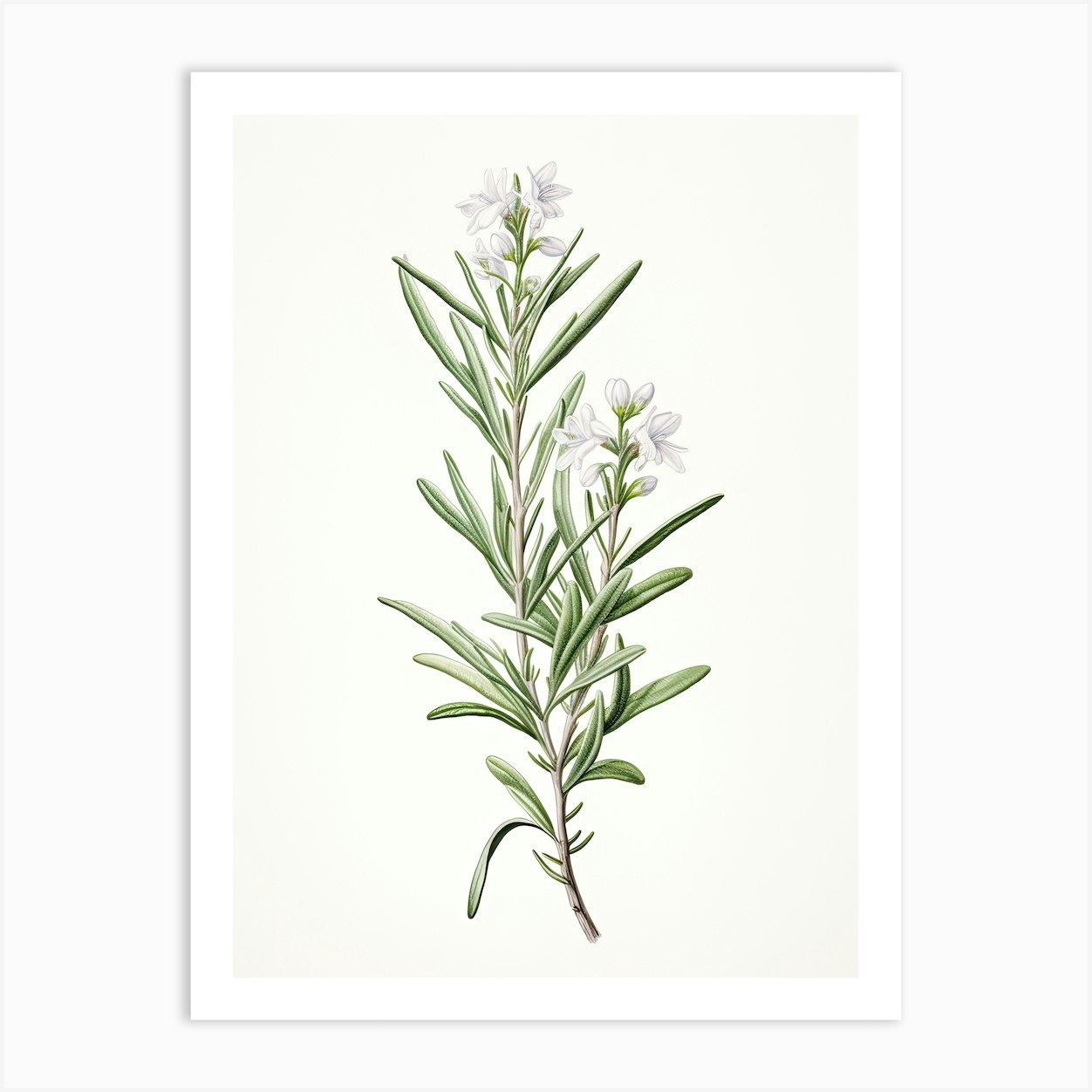This detailed color illustration, artistically rendered and portrait-oriented, showcases a botanical subject. The overall piece is vertically rectangular, framed with a thick white border and a narrow gray inner border, delivering a clean and minimalist presentation on what appears to be a fine cardboard canvas or a light cream background. The central focus of the illustration is a delicate plant with a single, straight stem that branches near the bottom into a smaller stem. Both stems bear clusters of white flowers at their tips. Some flowers are in full bloom, while others remain as buds. The plant features numerous light green, long, and tapered leaves accented with darker green lowlights, along with several shorter leaves also along the stem. The overall style is a photographic representationalism realism, capturing the botanical subject with intricate detail.